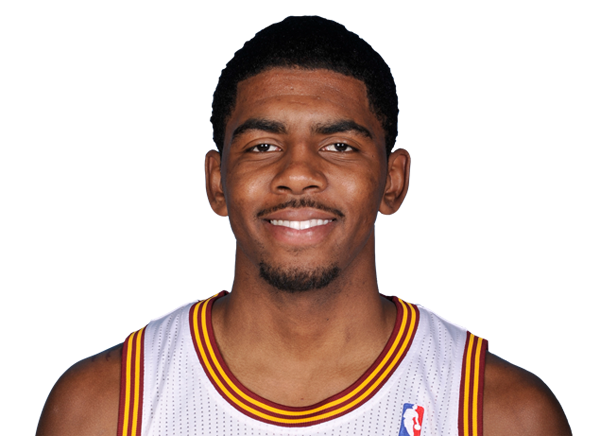This is a detailed photograph of an NBA player set against a plain white background, characteristic of a standard player profile photo. The player is a dark-skinned male with short, curly black hair, prominent eyebrows, a thin black mustache, and a small goatee on his chin. He is smiling cheerfully. He wears a white basketball jersey featuring red and gold trim around the collar and armholes, indicative of the Cleveland Cavaliers' color scheme. The jersey is perforated for breathability and displays the official NBA logo on the top left, a red, white, and blue insignia of a figure dribbling a basketball. The image captures him from the chest up, with no visible jewelry or other accessories, emphasizing his friendly and approachable demeanor.